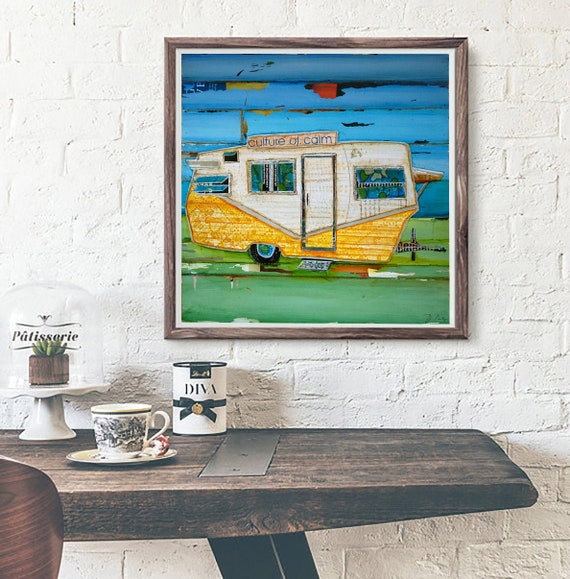The image captures a cozy interior scene inside a home, featuring a white painted brick wall as the backdrop. Hanging on this wall is a wooden-framed painting of a small camping trailer, distinguishable by its white and yellow color and single door, with the words "Culture of Calm" inscribed on it. Below the painting, an old wooden table is pushed against the wall, partially showing a wooden chair with a rounded back on the left-hand side. The table is adorned with a few items: a teacup and saucer, a canister labeled "Diva" with a black ribbon tied around it, and a cake display case with a transparent cover and white base, which may contain a dessert inside. Additionally, there's a wooden pot with a succulent plant sitting on another saucer or cake holder. The overall scene suggests a tranquil and inviting domestic space.